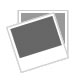The image appears to depict a minimalist graphic consisting of two overlapping squares resembling Polaroid photographs. The prominent square in the foreground features a dark upper portion, which is a deep, nearly black shade or possibly a very dark blue, contrasted by a thick white border around it and a notably thick white base at the bottom, akin to the classic Polaroid style. The second square in the background, partially obscured by the foreground square, presents a lighter grey shade and is similarly outlined by a white border. Both squares are positioned against a plain background, with the first one slightly angled to the right while the second maintains a straight alignment. The image is devoid of any text or additional colors, highlighting its simple, graphic nature.